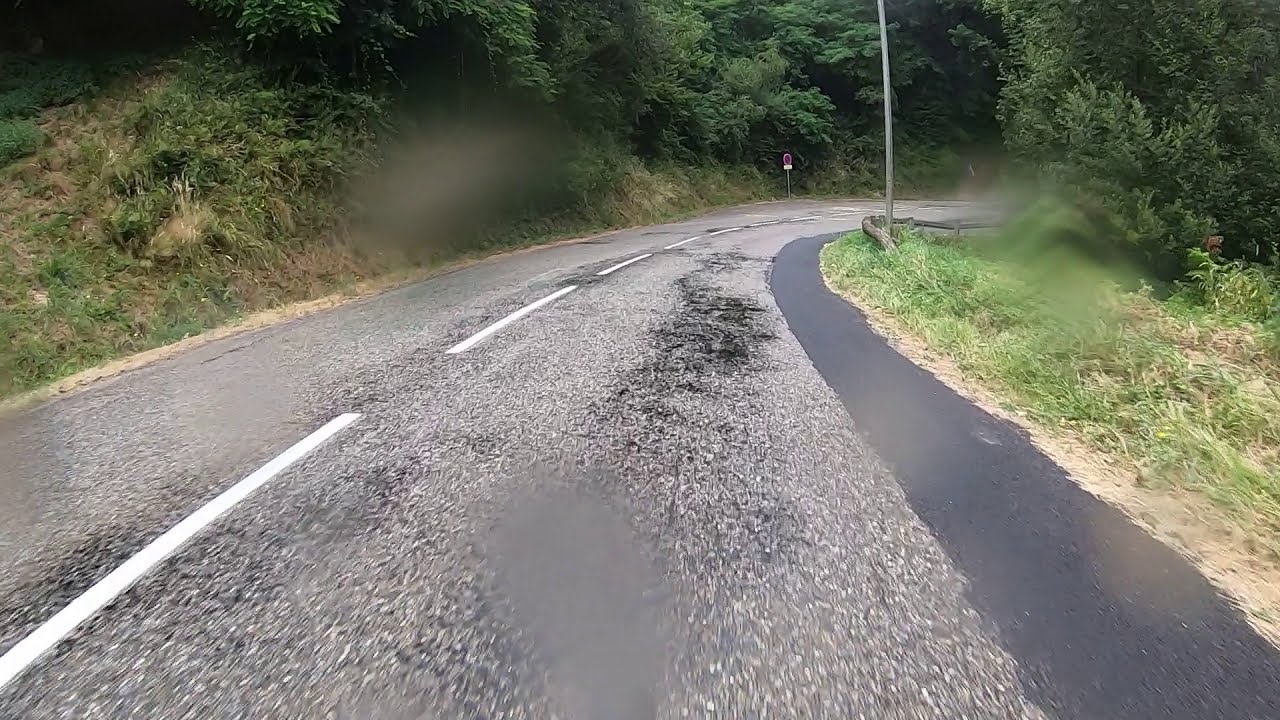This color, daylight photograph captures a wet, curving road in the middle of a lush forest. The road, made of gray and black asphalt, is divided by white dotted lines and shows signs of some damage with small holes on the surface. Patches of the road appear darker due to recent rainfall, and raindrops can be seen on the camera lens, causing parts of the image, particularly the bottom and upper edges, to appear blurred. The road, featuring two lanes, disappears to the right around a bend and is bordered by green grasses and dense trees. On the right side of the road, the foliage is a mix of green and brown, with tall trees standing further back. In the distance, a wooden rail and a blue and red traffic sign are visible. To the left, the ground rises sharply, covered with tall, dark green trees and thick, natural vegetation, creating a sense of an enclosed, natural setting.